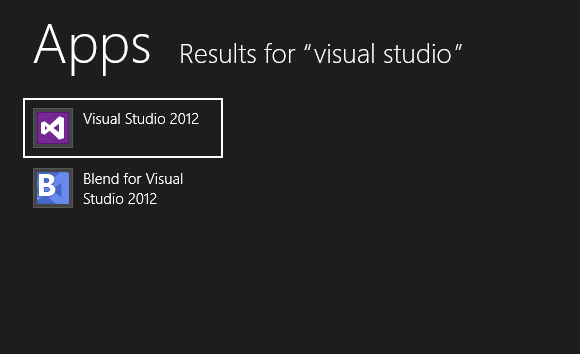The image portrays a Windows search bar within the taskbar, wherein a user has typed "Visual Studio." The search results are displayed against a black background with contrasting white text. Two specific results are visible: "Visual Studio 2012" and "Blend for Visual Studio 2012." The first result, "Visual Studio 2012," is highlighted with a box around it, suggesting it might be the default selection or about to be selected by the user. Both results feature HTML icons. The Visual Studio icon resembles a three-dimensional hourglass, angled in a way that makes one end appear closer to the viewer. The Blend icon is similar but includes a prominent 'B' to designate Blend. The juxtaposition of the two icons and the user interface adds clarity to the Visual Studio suite options available.